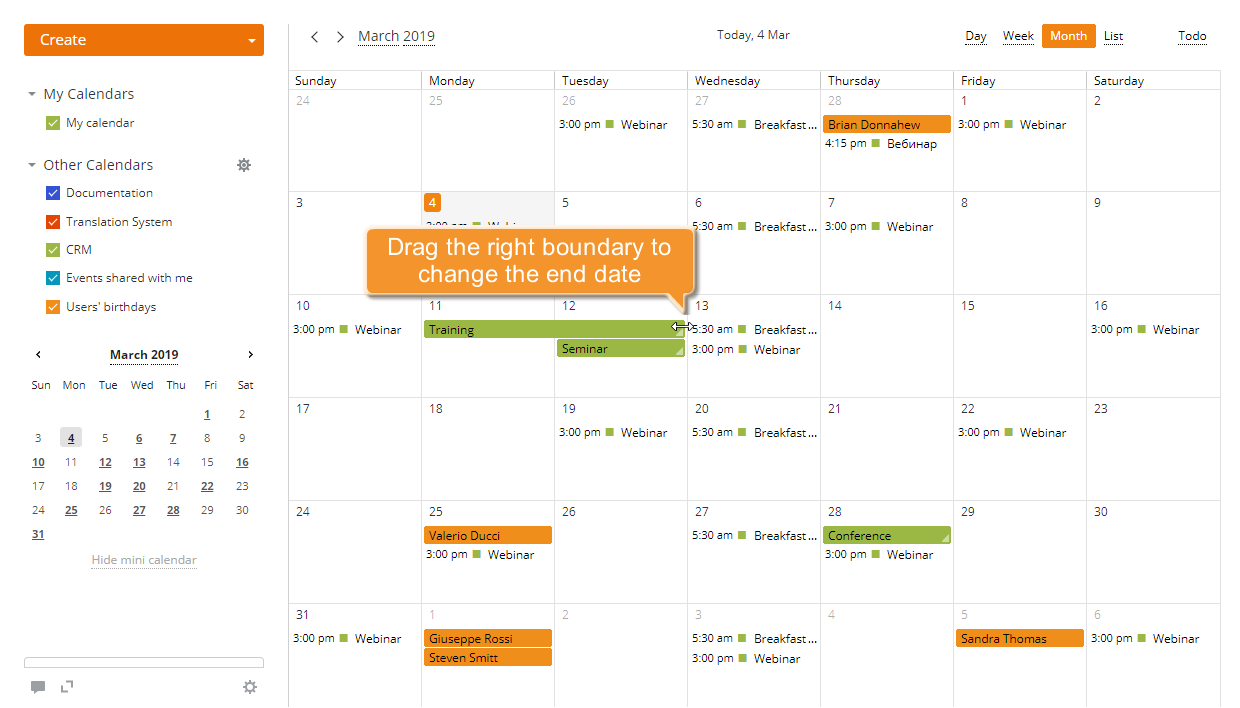The image depicts a digital calendar interface from March 2019, likely viewed through some calendar management software. On the left side of the screen, there is a navigation pane labeled "My Calendars" and "Other Calendars," listing various calendar categories such as "Documentation," "Translation System," "CRM," "Events Shared with Me," and "Users’ Birthdays," all of which are currently enabled. 

The main calendar display features a month view with a specific focus on March 4th, although this date is partly obscured by an informational pop-up. Notably, a new event titled "Training" was recently added for March 11th and has been extended to span two days, ending at the conclusion of March 12th. A tool-tip at the event’s boundary indicates that the end date can be adjusted by dragging. The cursor is represented by a double arrow, allowing the user to modify the event's duration. 

Throughout the calendar, there is a multitude of scheduled events, with many being related to birthdays, highlighting an active and event-filled month.